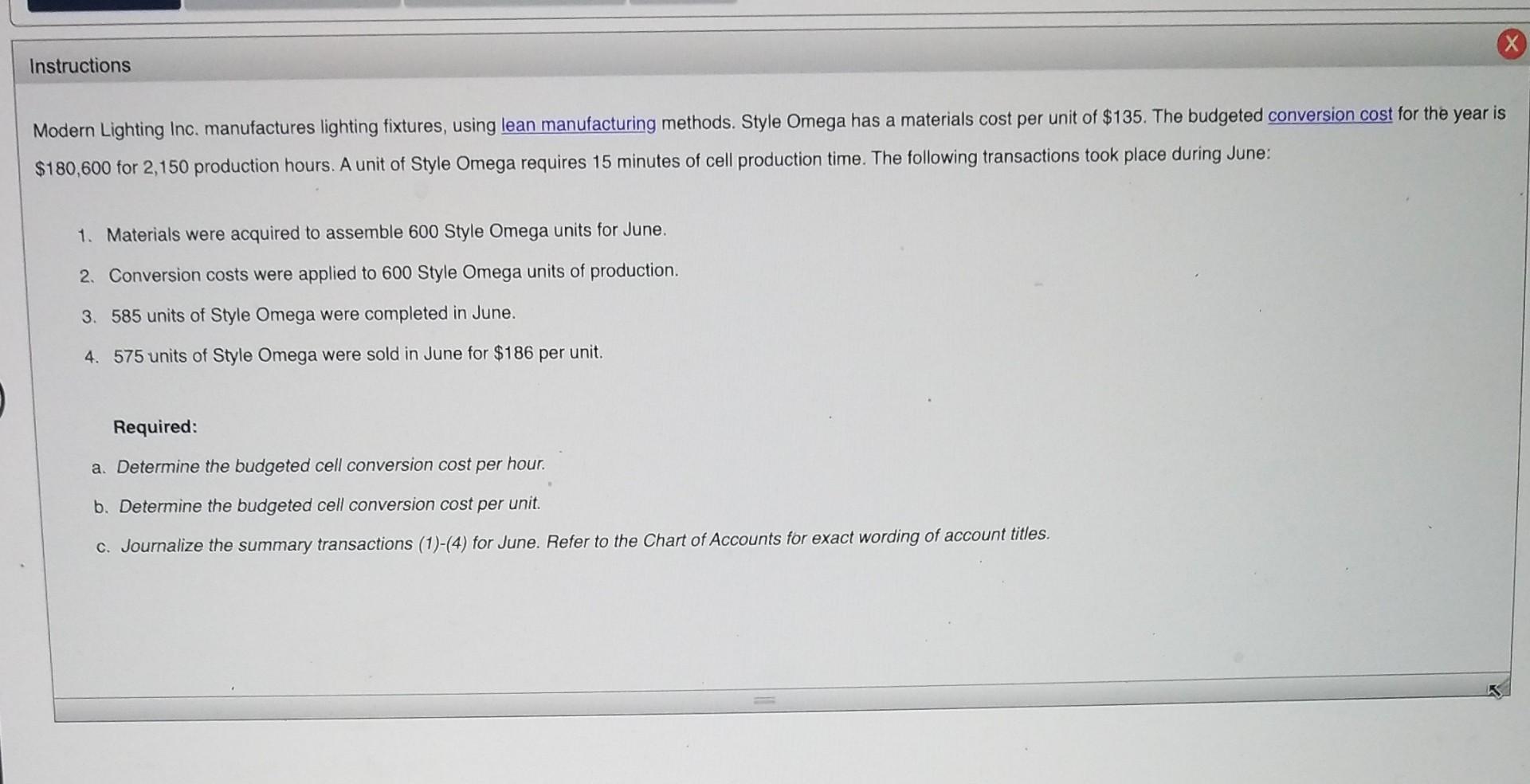The image displays a screenshot from a website with a predominantly white background. At the top, there is a light gray banner featuring the word "Instructions" in black text. Below this banner, the following text is presented:

---

**Modern Lighting, Inc.**  
Manufacturers of lighting fixtures using lean manufacturing methods. 

*Lean manufacturing* (underlined and in blue text)

---

The detailed information reads:

---

**Style Omega has a material cost per unit of $135.**

**Budgeted conversion cost for the year: $180,600 for 2,150 production hours.**  
Each unit of Style Omega requires 15 minutes of production time.

---

**June Transactions:**
1. Materials were required to assemble 600 Style Omega units for June.
2. Conversion costs were applied to 600 Style Omega units of production.
3. 585 units of Style Omega were completed in June.
4. 575 units of Style Omega were sold in June for $186 per unit.

---

**Required:**

A. Determine the budgeted conversion cost per hour.  
B. Determine the budgeted conversion cost per unit.  
C. Journalize the summary transaction (transactions 1 to 4 for June), referring to the chart of accounts for exact wording of account titles.

---

Both "lean manufacturing" and "conversion cost" are underlined and highlighted in blue text.